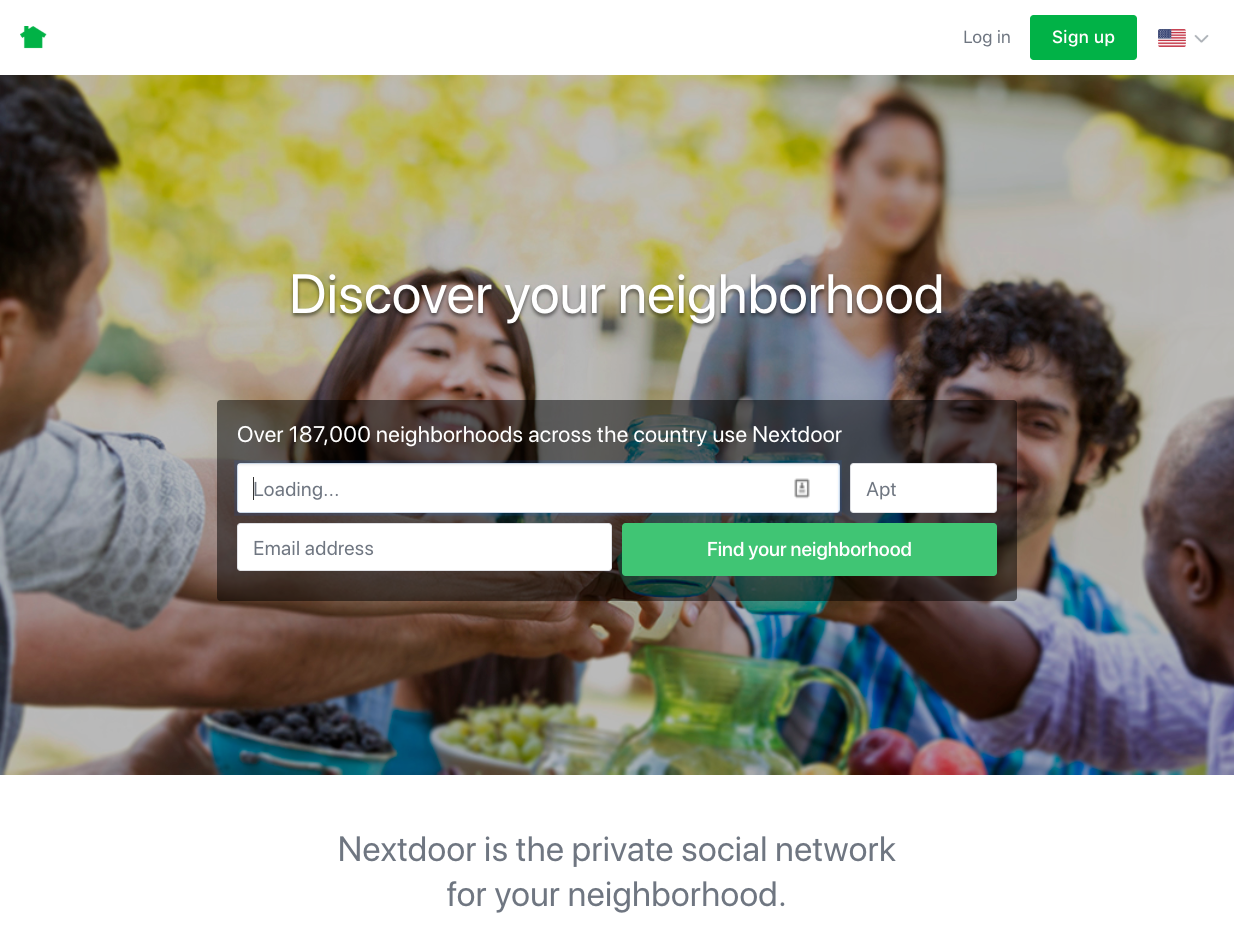This image captures a warm, community-centric scene. In the foreground, a group of diverse individuals comprising two men and two women are seen gathered around a table laden with fresh fruits such as apples, peaches, a bowl of blueberries, and grapes. A clear, green glass pitcher sits prominently on the table. The background is slightly muted, featuring what appears to be trees.

Among the people, an Asian girl faces the camera, while another girl and an Afro-American man with curly black hair are partly visible in the background. The photo exudes a sense of togetherness and neighborhood camaraderie.

Overlaying this scene, a translucent black banner contains several informative texts: 
1. At the top, "Over 187,000 neighborhoods across the country use Nextdoor."
2. In the middle, the invitation "Discover your neighborhood."
3. Below this, there are multiple banners: a white banner reading "Loading," another that says "APT" (likely indicating 'apartment'), a space for "Email address," and a green banner urging action with "Find your neighborhood."

In the top right corner, there are options for account management: a "Log in" button and a green "Sign up" button. Adjacent is a small US flag icon with a downward pointing arrow, suggesting the potential for region or language change.

On the far left, a green house icon outlines the thematic focus of the application. 

Below the image, the description reads: "Nextdoor is the private social network for your neighborhood." This tagline emphasizes the private and localized nature of the Nextdoor platform.